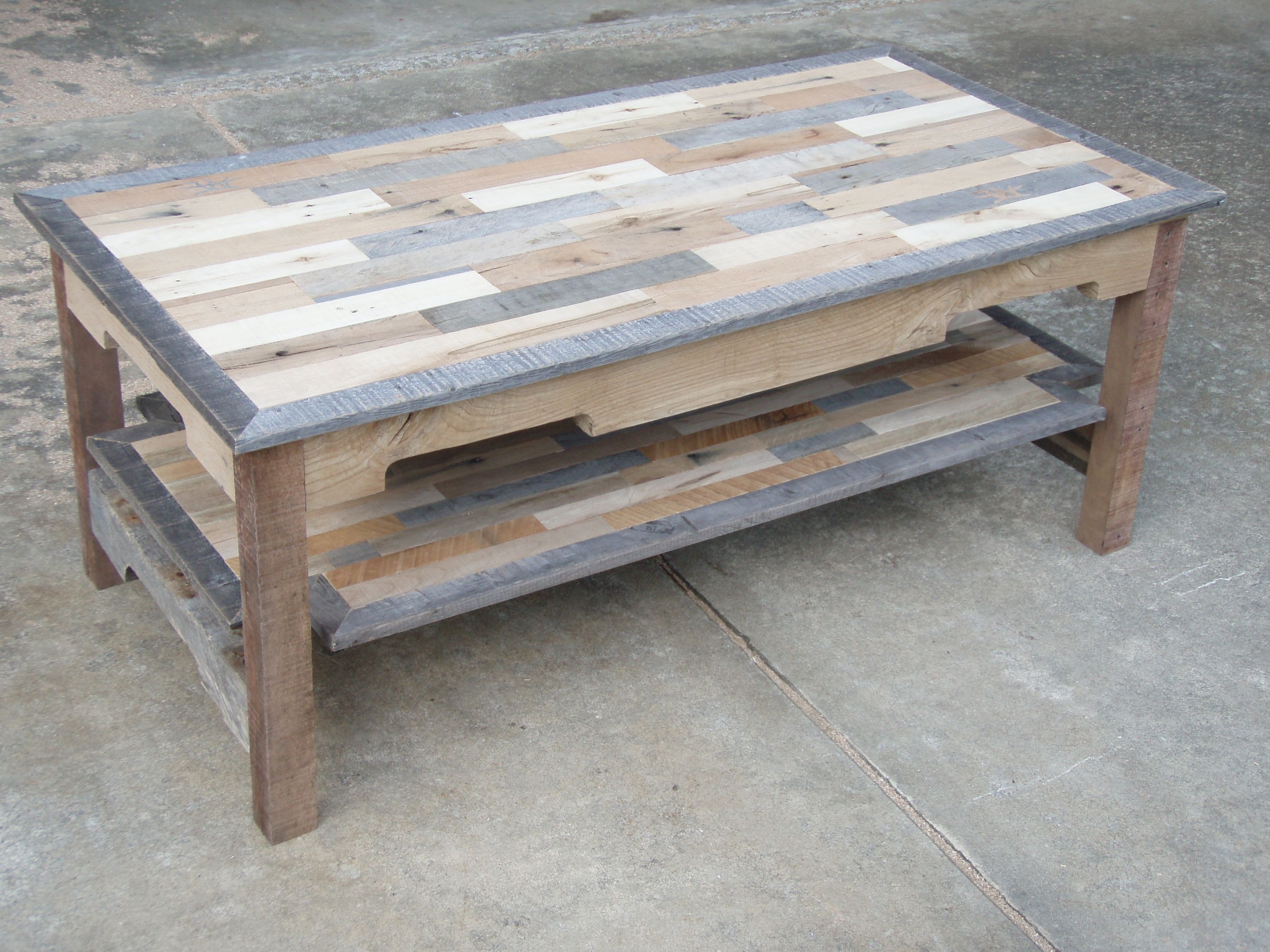In this color photograph, a handmade, intricate coffee table is positioned outdoors on a concrete or paved surface. The table showcases a distinctive blend of multiple types of wood, arranged in a visually striking and detailed pattern. The top surface of the table is composed of various wood tones, including light brown, very light almost white wood, darker wood, gray wood, and some pieces with gray and brown knots. The legs of the table are made of a darker wood, possibly burl wood, adding to its rustic charm. Additionally, the table features a lower shelf constructed from the same multicolored wood pieces as the top, enhancing its practicality and unique aesthetic. The table’s eclectic mix of wood colors and textures gives it a quirky and appealing appearance.